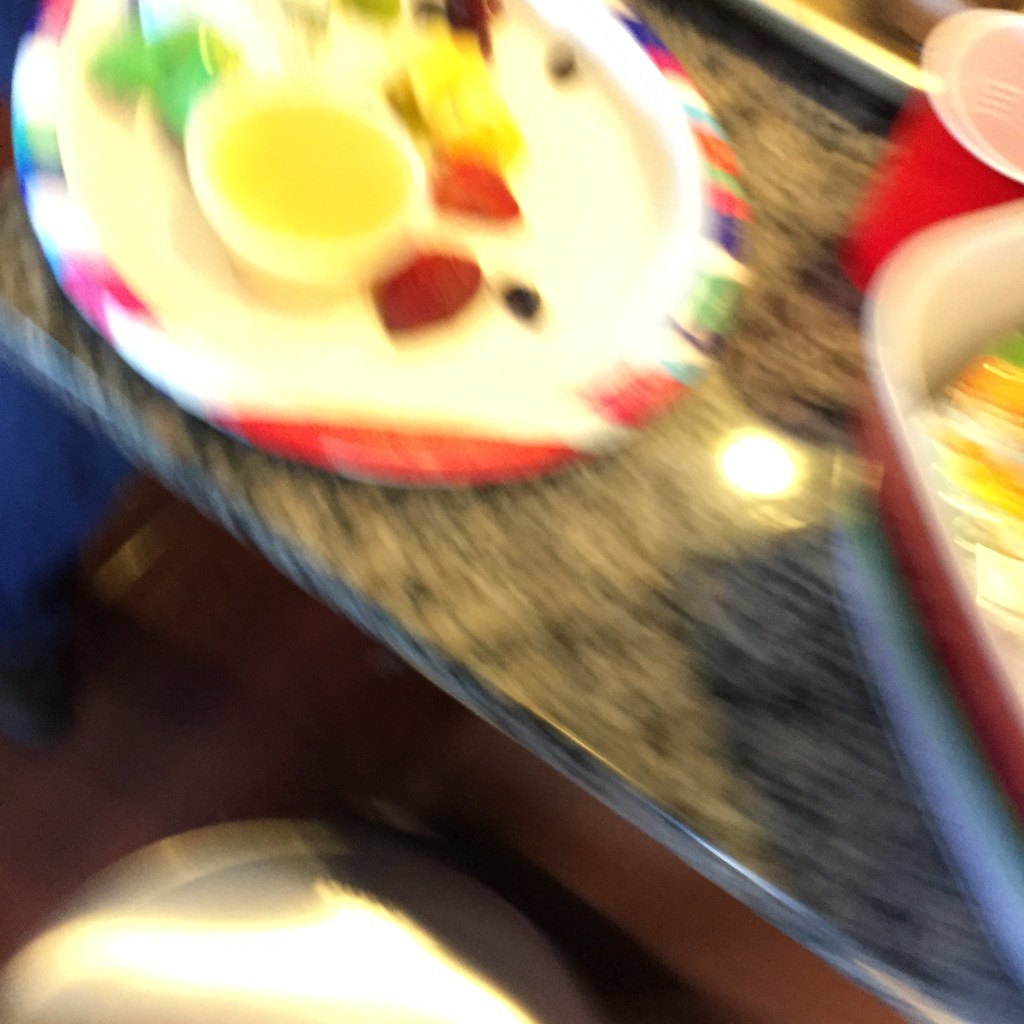The image is a blurred, vibrant color snapshot taken from an overhead perspective, capturing a scene on a granite countertop. The countertop, bathed in bright light from an unseen source slightly right of center, showcases a paper plate filled with vividly colored, though somewhat indistinguishable, food items. Positioned near the center-right of the image is a casserole dish, partially visible, with a distinctive red solo cup situated just behind it. The shelf or table on which these items rest appears to be aligned diagonally, spanning from the top left to the bottom right corner of the photograph. On the floor below, there is an indistinct white circular object reflecting the overhead light, adding to the overall brightness and vivid coloration of the scene.